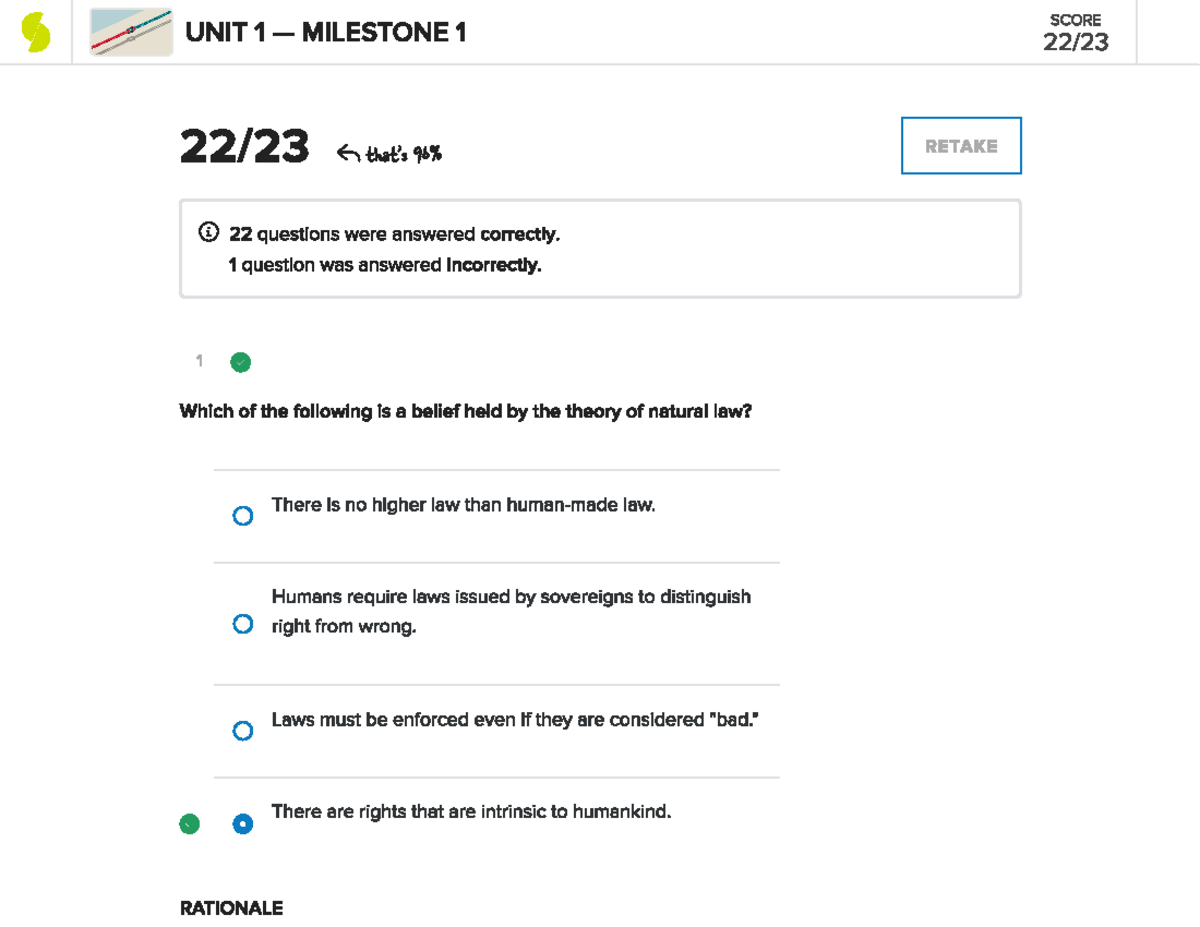A detailed and cleaned-up descriptive caption for the image could be:

"This image features a learning dashboard, possibly from an educational platform. In the top left corner, there is a circular icon divided in half, with the left half colored red and the right half blue, resembling a pulley. Adjacent to the icon, in bold black text, is the title '1 - Milestone 1'. To the right of the title, it indicates a score of '22 out of 23' in smaller text, with the larger text below emphasizing the score as '22 out of 23' and specifying '96%' in black text. 
  
In the same area, there is a blue-bordered box containing the word 'Retake' in grey text. Below this section, there appears to be an information bubble icon. The text reads '22' in bold, followed by 'questions answered correctly' indicating perfect correctness for 22 questions. Underneath, it mentions that '1 question was answered incorrectly,' marked with a green checkmark to the right.

The question displayed below the score summary is: 'Which of the following is a belief held by the theory of human law?' Four answer choices are provided in blue colored bubbles. The three unselected options are: 
1. 'There is no higher law than human-made law.'
2. 'Humans require laws issued by sovereigns to distinguish right from wrong.'
3. 'Law seems to be enforced even if they are considered bad.'

The correct answer, distinguished by a green checkmark to its left, reads: 
'There are rights that are intrinsic to humankind.' 

At the very bottom, there is a section labeled 'Rationale' presumably meant to provide further explanation or justification for the answer."